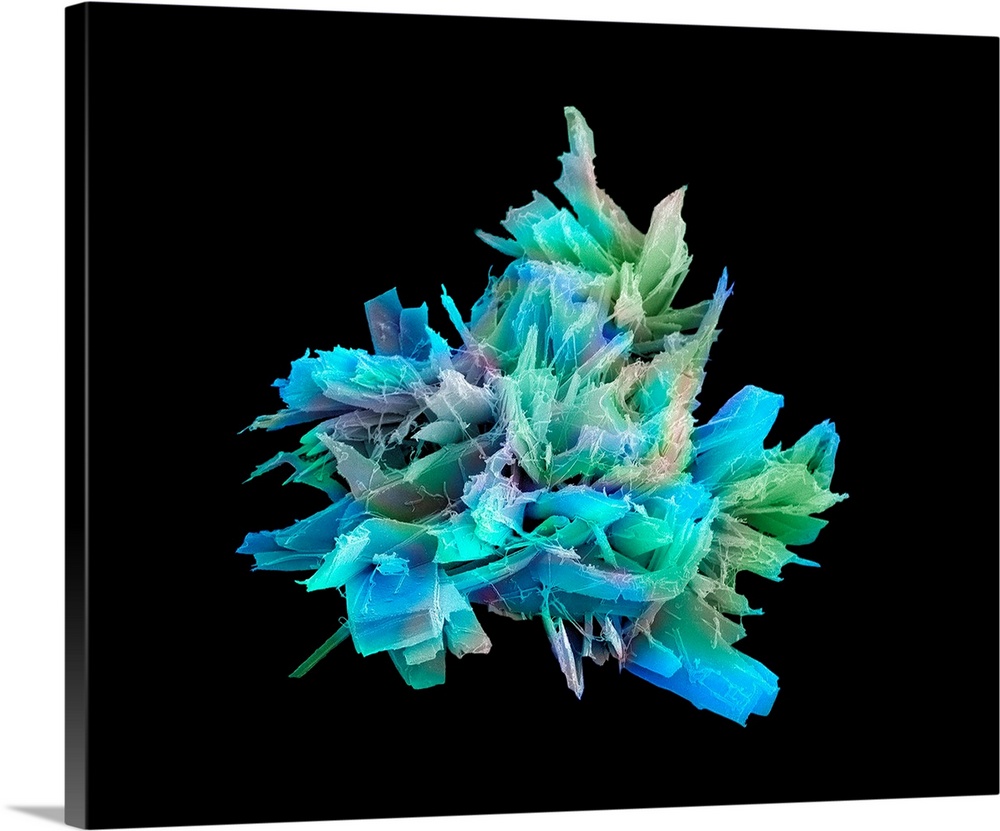The image is a detailed piece of art printed on a rectangular canvas with a rich black background that wraps around the wooden frame. At the center of the canvas, occupying about half of the total area, is a striking three-dimensional structure resembling an intricate, zoomed-in photograph possibly taken with a scanning electron microscope. The centerpiece of the artwork features a jagged, pointy structure that gives the impression of sharpness, as if touching it could cause a cut. This vivid central object displays a spectrum of colors, including bluish-green, purple, and touches of peach, contributing to an overall ethereal appearance reminiscent of an oceanic reef under a glow-in-the-dark effect. The structure appears to have multiple ridges and irregularities, and shadows are cast, particularly noticeable in the bottom left corner of the image. The canvas itself contains no text, allowing the viewer to fully engage with the mesmerizing, high-level details of the piece.